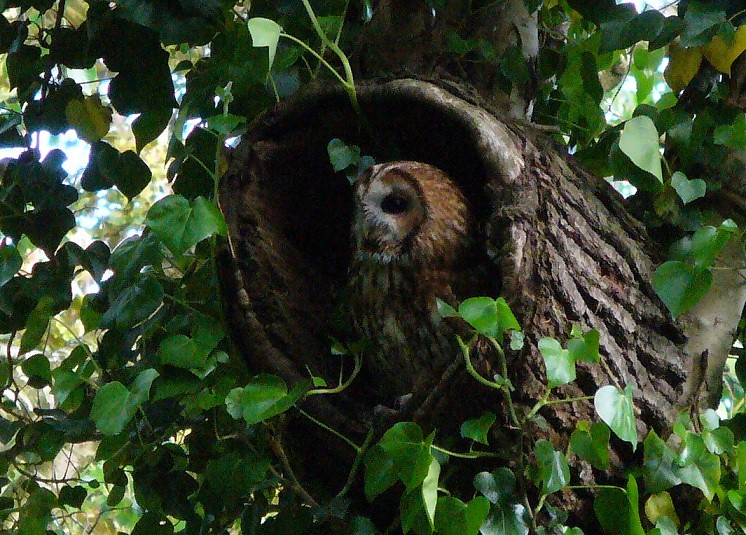In the bright, sunny forest, an oak tree, thick with bark and adorned with lush green leaves and ivy, stands prominently. Among the foliage, a large knot hole or hollowed-out branch draws attention. Nestled within this natural cavity is a barn owl, with its brown and white plumage artfully contrasting against the tree's rough texture. The owl's face, predominantly white with brown feathers forming a widow's peak down its front, features striking black eyes and a yellow beak, with hints of red around the beak suggesting a recent meal. Through gaps in the leaves, patches of blue sky and distant trees are visible, adding depth to the serene woodland scene.